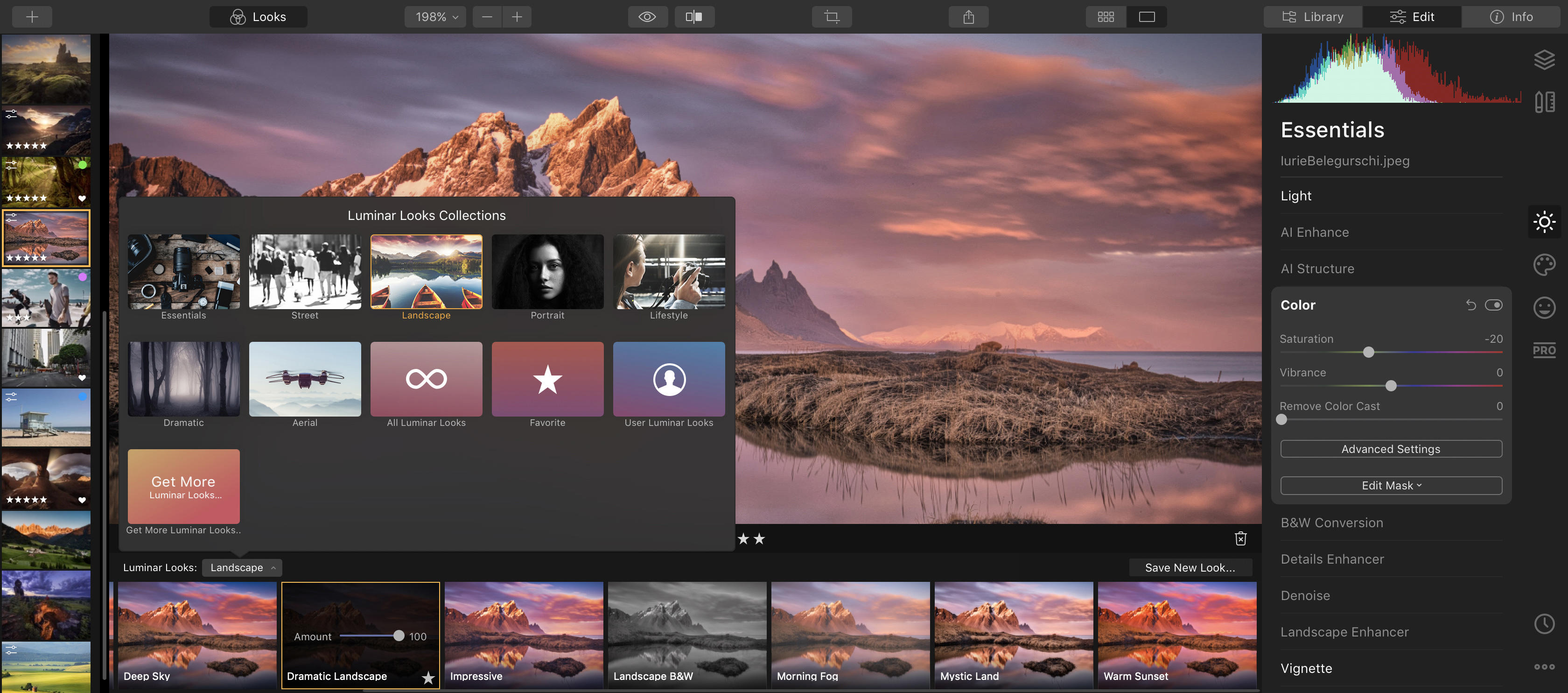This image, sourced from a website, depicts a stunning outdoor scene with prominent natural features. In the background, majestic mountain peaks are visible, although partially obscured by a pop-up window on the screen. The landscape includes a blend of land and water, with the setting sun casting a mesmerizing palette of gray and pink hues across the clouds. These colors are beautifully reflected in the water below, accompanied by patches of green grass.

At the center of the image, a pop-up showcases various photographs under the theme of celebrations, though the text is too small to read clearly. This pop-up includes a maroon-colored button inviting viewers to "Get More" images. Along the left edge of the main image runs a vertical column of photographs, enhancing the visual appeal.

On the right side, labeled as "essentials," is an interface with several interactive elements. This includes a colorful graph with segments in white, purple, maroon, green, and blue, documenting features labeled AI-enhanced and AI-structure. Additionally, there is a section dedicated to color adjustments, complete with sliders that users can manipulate to customize the image further. This interface box is presented in a sleek black design, adding a modern touch to the overall visual experience.